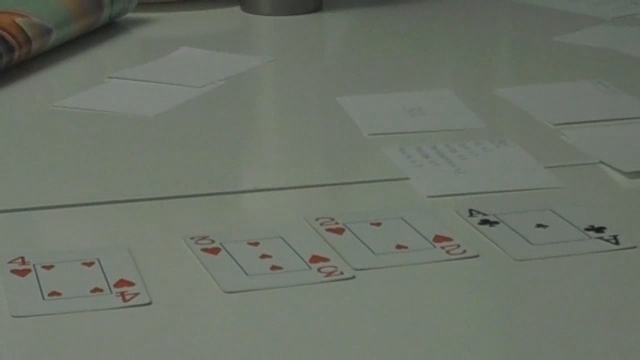In this slightly out-of-focus and poorly lit color photograph, a cluttered white or light-colored table serves as the setting. The top left corner of the table features a partially visible, rounded edge of what appears to be a folded or rolled magazine. Adjacent to this, two sheets of blank white paper lay flat. At the center of the top edge of the photo, a conical bottom of an item, possibly a mug or a coffee carafe, can be discerned. The top right corner holds additional white pieces of paper. Halfway down the right side of the table, more sheets of white paper are visible.

Dominating the middle of the table are two white pieces of paper, one displaying a small amount of writing and the other bearing more extensive notations, accompanied by a pencil. Spread across the bottom portion of the table are four face-up playing cards: the four of hearts, the three of hearts, the two of hearts, and the ace of clubs. The playing cards are simple and not elaborately adorned.